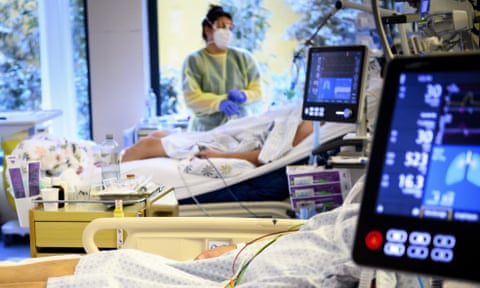The photograph depicts a hospital room with two patients lying in hospital beds wearing blue and white gowns. Their faces are obscured by complex medical machinery. One patient is positioned in a more elevated bed with their head raised, and their bare legs, arms, and shoulders visible. The room’s walls are white, and large windows reveal a lush green view of numerous plants and trees outside. Between the two beds, there are purple packages and various trays with medical supplies. Both beds are yellow, and each has monitoring devices attached with blue displays showing unclear white text. Though the numbers 30, 30, 52, and 143 are visible on the closer machine, the readings on the other are indistinguishable due to blur and distance. In the background, a medical personnel, possibly a doctor or a nurse, is seen wearing light blue scrubs, a white surgical mask, and bluish purple gloves. They appear to be examining or monitoring one of the patients.